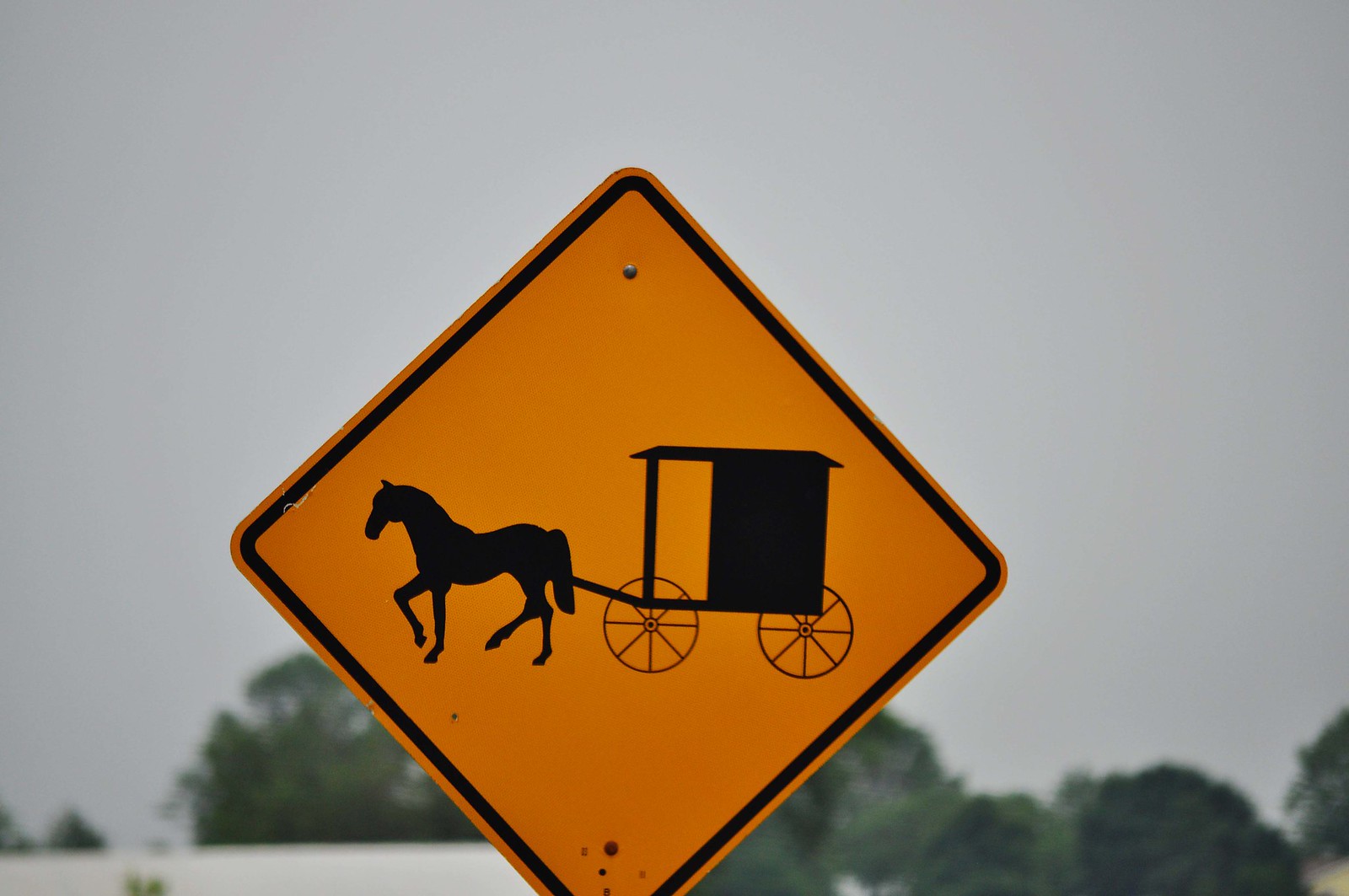In the image, there is a cautionary street sign prominently featured in the center. The sign is diamond-shaped with a yellowish-orange background and a distinct black border framing it. Inside the sign, there is a black silhouette illustration of a horse, which is positioned on the left side, walking towards the left. Attached to the horse is a long stick-like harness connected to a small carriage. The carriage is depicted as a black box-like structure with a roof, and it features a small white section on the right side, which appears to be a door. The carriage is supported by two large wheels, each with eight visible spokes. 

The background of the image is slightly blurred, with a grayish-blue sky above and the tops of trees near the bottom of the frame. The bottom left corner of the image shows a patch of white, possibly reflecting light or another element. Overall, the image captures the essence of a traditional horse-drawn carriage sign against a soft, muted natural backdrop.